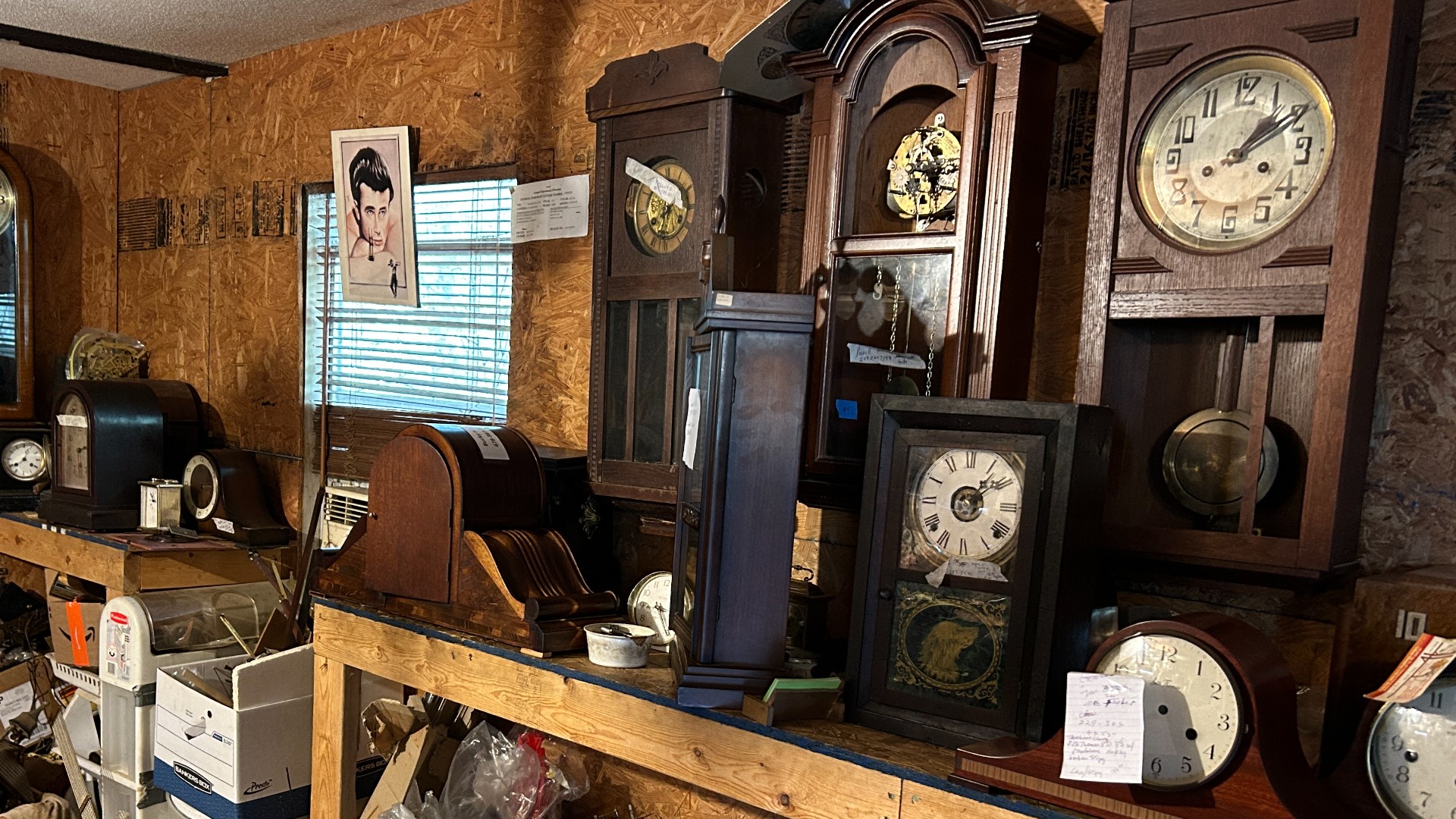The image appears to be taken inside a probable antique or secondhand store featuring a substantial collection of wooden clocks. These antique timepieces, with their old, time-worn, weathered faces, are the primary focus, displayed prominently on two wooden shelves. One shelf is positioned in the left corner, extending diagonally towards the left side of the image from the lower right corner, while the other shelf is in the right corner. Both shelves are crowded with a variety of clocks, including wall-mounted, mantel clocks, and freestanding ones, in an array of wood tones from deep and lighter browns to almost blackish shades.

The background wall, made of unfinished particle board, further emphasizes the rustic and vintage ambiance of the setting. Between the two shelves, a window with mini blinds is visible, adorned with a picture of James Dean hanging over it. The lower parts of the shelves feature storage compartments cluttered with various items, boxes, and racks, contributing to the untidy yet charming atmosphere typical of such stores. The floor beneath the shelves is scattered with miscellaneous items, adding to the eclectic and historical feel of the room.